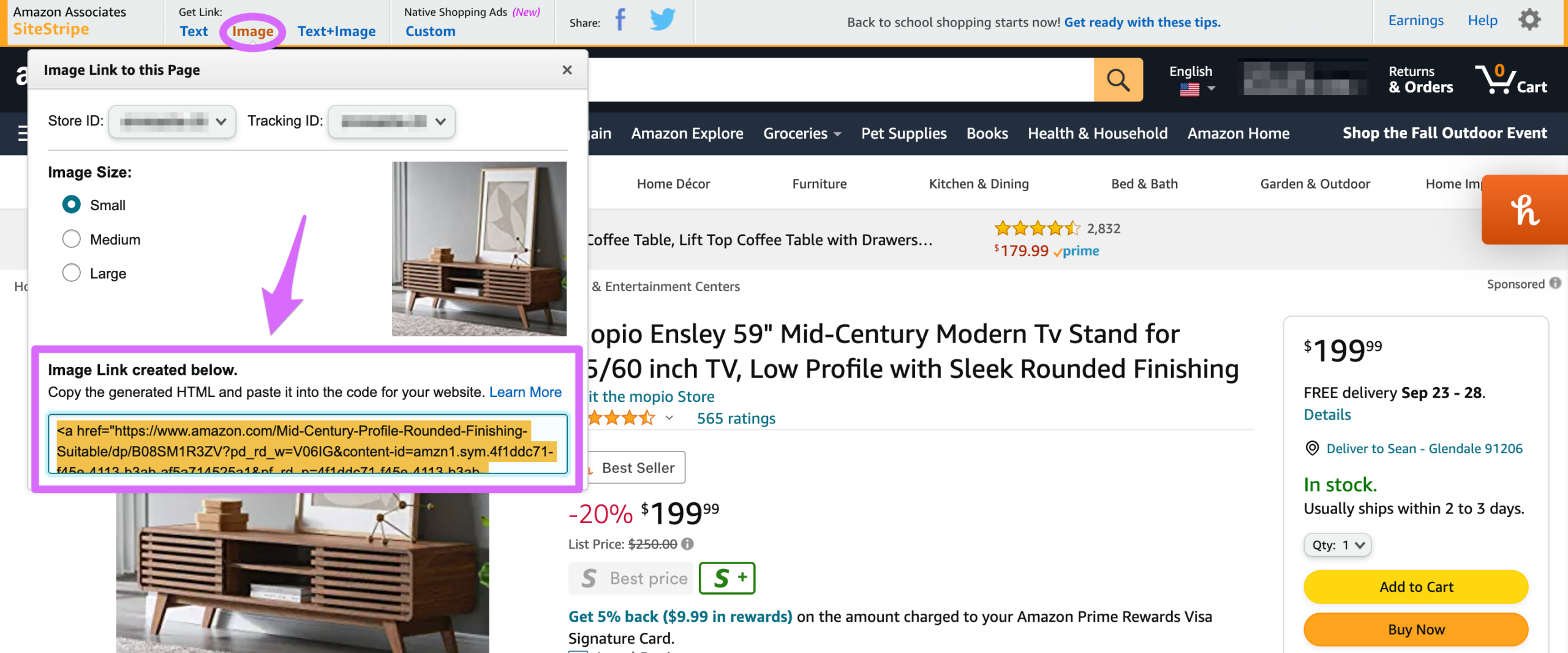The image showcases an Amazon product page, enhanced by an Amazon Associates site stripe above the typical Amazon layout. The stripe includes a left-aligned label reading "Amazon Associates Site Stripe," followed by a "Get Link" section comprising options for text, image, and text+image links. The "Image" option is specifically circled in purple.

In the forefront, a pop-up box partially covers the Amazon product page. The top of this pop-up reads, "Image link to this page," with a store ID and tracking ID that are redacted. The pop-up displays an image identical to the one on the Amazon product page, depicting a modern TV stand. To the left of this image, there are options for image sizes: small, medium, and large, with the "Small" size circled.

A purple arrow points to the bottom of the pop-up window, which instructs, "Image link created below. Copy the generated HTML and paste it into the code for your website." Below this instruction, the generated HTML code is highlighted in orange and enclosed in a lilac box for emphasis.

The Amazon product page in the background lists the TV stand priced at $199.99 with free delivery estimated between September 28th and September 28th. The item is indicated to be in stock and typically ships within two to three days. The page features a distinctive yellow "Add to Cart" button and an orange "Buy Now" button beneath it.